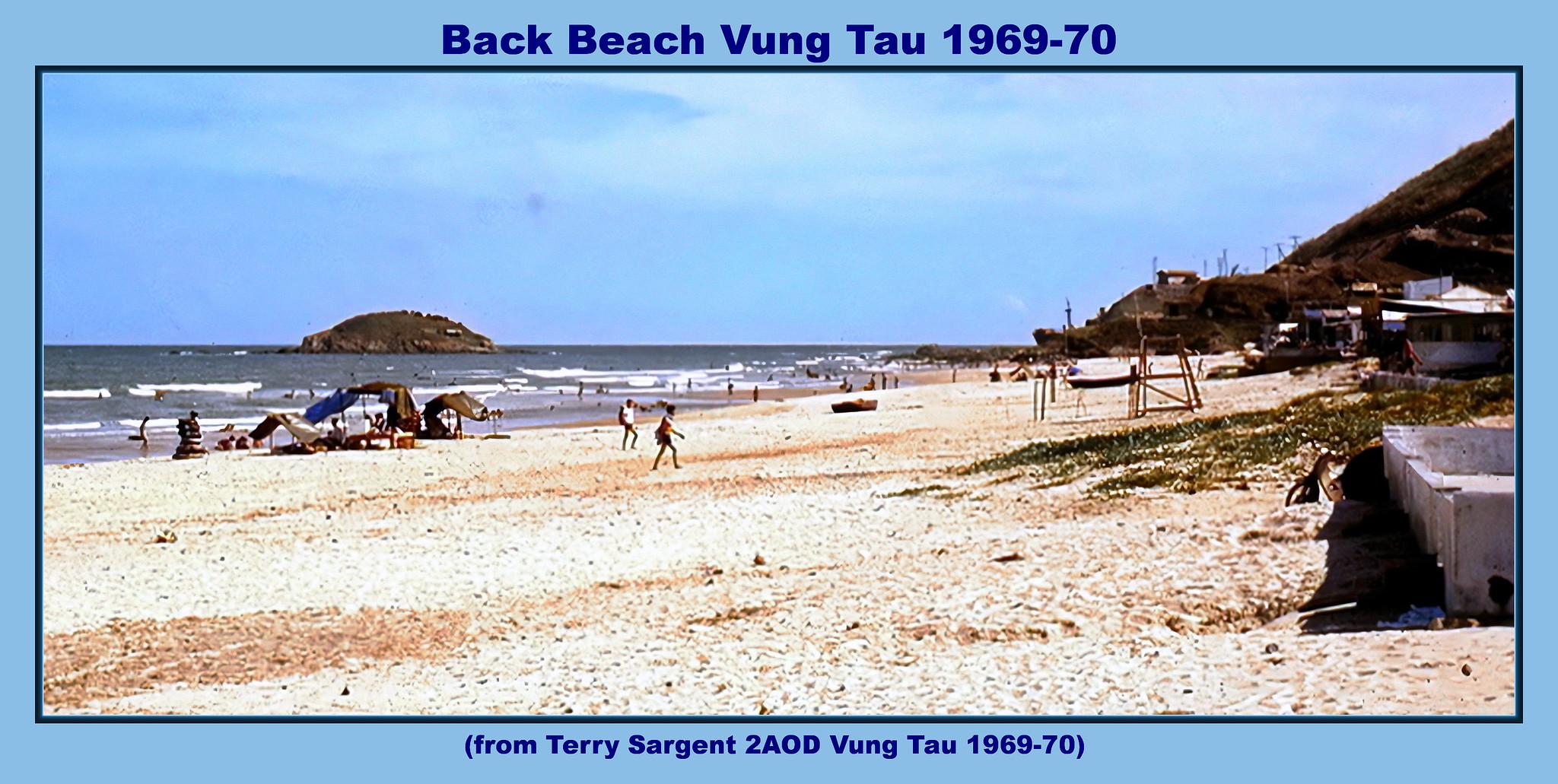The image resembles an old postcard with a light blue border and a black inner border. The top of the postcard features blue text on a light blue background that reads, "Back Beach Vung Tau 1969-70." At the bottom, it is inscribed in the same blue text, “From Terry Sargent to AOD, Vung Tau 1969-70.” This seaside photograph captures a sandy beach in Vung Tau, Vietnam, dating back to the Vietnam War era.

The beach is depicted under a sky that transitions through various shades of blue and white with some clouds. The sand's colors range from light yellow to dark brown, and there are sparse patches of grass, particularly on the right side of the image. Dotted across the sandy expanse are numerous small figures of people, either enjoying the shoreline or wading into the ocean. In the background, on the right, there are small huts and dilapidated buildings, indicators of a war-torn setting rather than a typical tourist destination.

The ocean itself stretches across the left and center of the photograph, with gentle waves breaking on the shore. There is a small island or mound visible in the distant ocean, adding to the scenic, albeit stark, wartime atmosphere. Farther right in the backdrop, hints of a cropped mountain range or hills can be seen. The subdued tones and the orderly composition provide a glimpse into life during that historical period, balancing the natural beauty of the beach with the underlying melancholy of its wartime context.